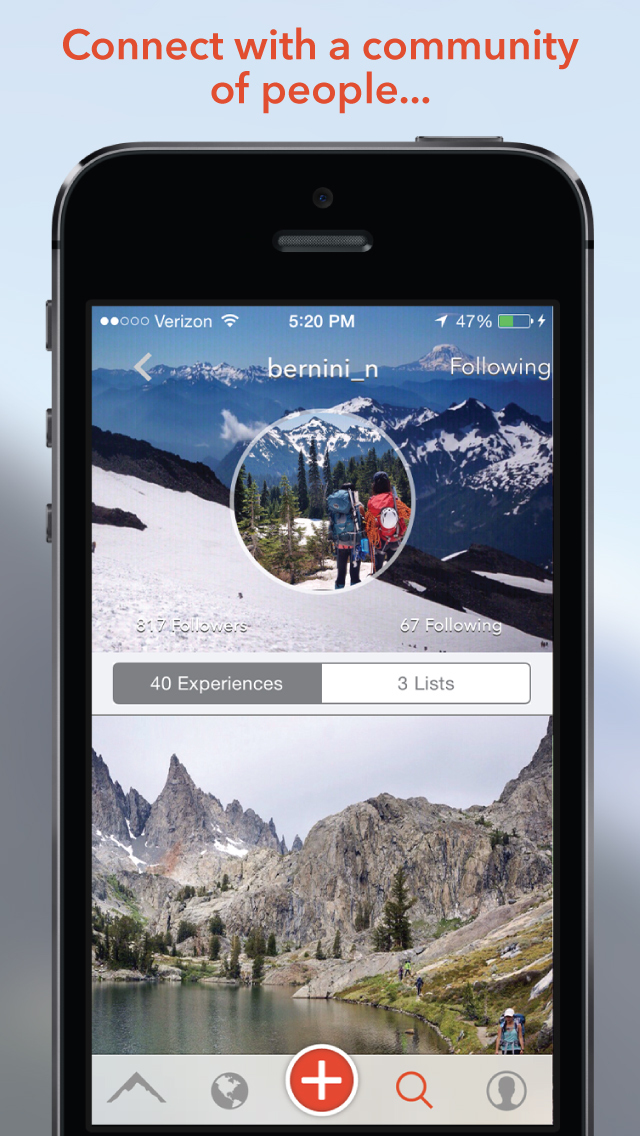The digital screenshot illustrates a vibrant scene centered around community interaction. Dominating the image is a large, photoshopped cell phone, prominently displaying a Verizon logo at the top of its screen. The screen shows full connectivity with five filled white dots, as well as the Wi-Fi bars and the current time of 5:20 PM. The battery indicator suggests varying levels: 40% and 47%.

On the screen, a user named "Nini_in" is shown, alongside a notification indicating new followers. Behind this digital setup, the backdrop showcases a picturesque wilderness setting with two individuals. These adventurers, dressed warmly with backpacks, are surrounded by trees and snow-capped mountains, signifying a wintery environment. Below the image, Nini_in's profile statistics are highlighted: 317 followers, 67 following, 40 experiences, and 3 lists. The entire composition underscores the theme of connecting with a like-minded community amidst natural beauty.